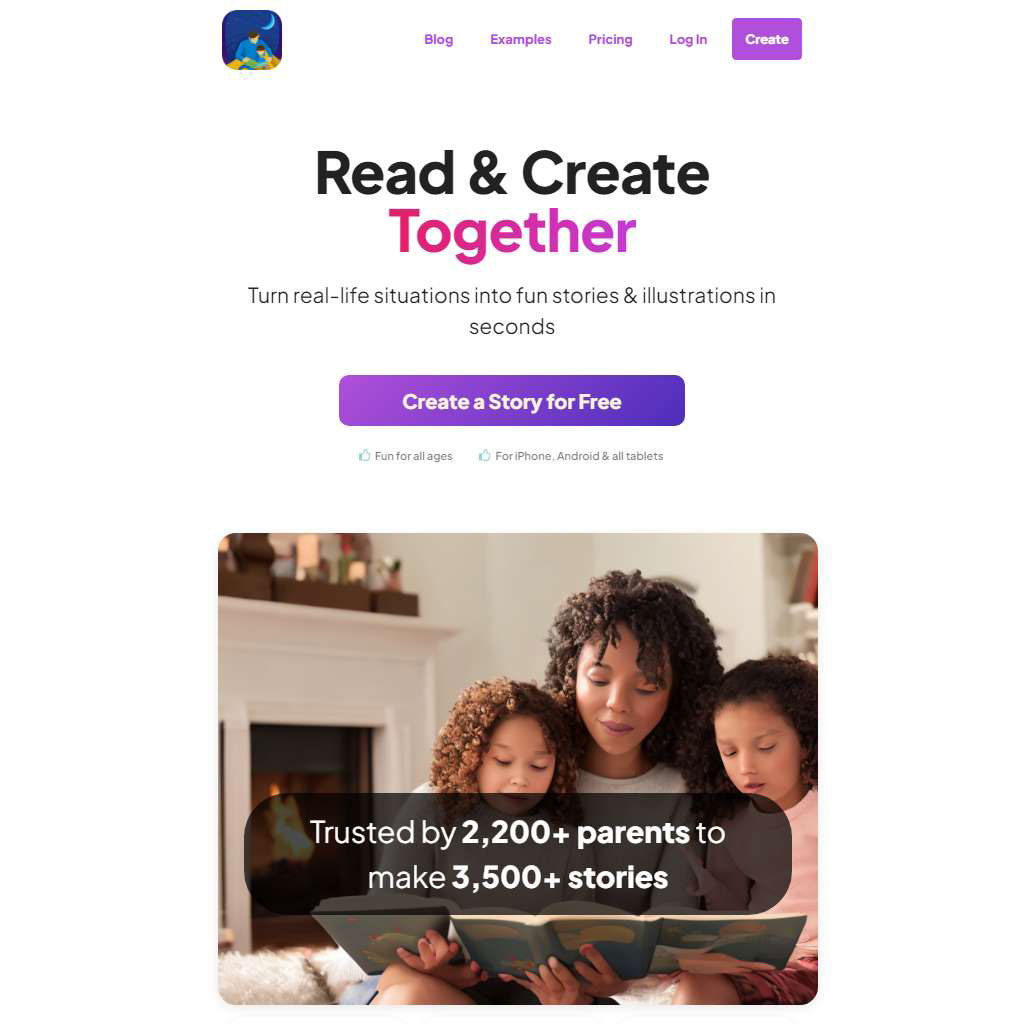The image features a white rectangular layout with no borders, creating a floating effect for the various elements arranged within it. 

In the upper left corner, there is a small blue cartoon icon depicting a man reading to his son against a backdrop of a blue sky and a crescent moon. Running across the top of the layout in small purple print are the navigation links: "Blog," "Examples," "Pricing," and "Login." In the upper right-hand corner, a prominent "Create" button is displayed.

About halfway down the layout, the text "Read and Create" appears in black font, followed by "Together" in a gradient large font transitioning from light red to purplish. Below this, a small black font describes the service: "Turn real-life situations into fun stories and illustrations in seconds." 

There is a purple box beneath this text, featuring white lettering that reads, "Create a story for free." Below the box is additional information in smaller text: "Fun for all ages, for iPhone, Androids, and tablets."

Towards the bottom of the layout, there is a heartwarming picture of a woman in her 30s reading to her two daughters, who appear to be around 8-10 years old. They are seated in front of a fireplace with a white wall and a mirror above it. A transparent black box with white text overlays the image, declaring, "Trusted by 2,200+ parents to make 3,500+ stories."

In essence, this visually compelling and detailed layout captures the essence of a platform designed to bring families together through storytelling, ensuring fun and creativity for all ages.